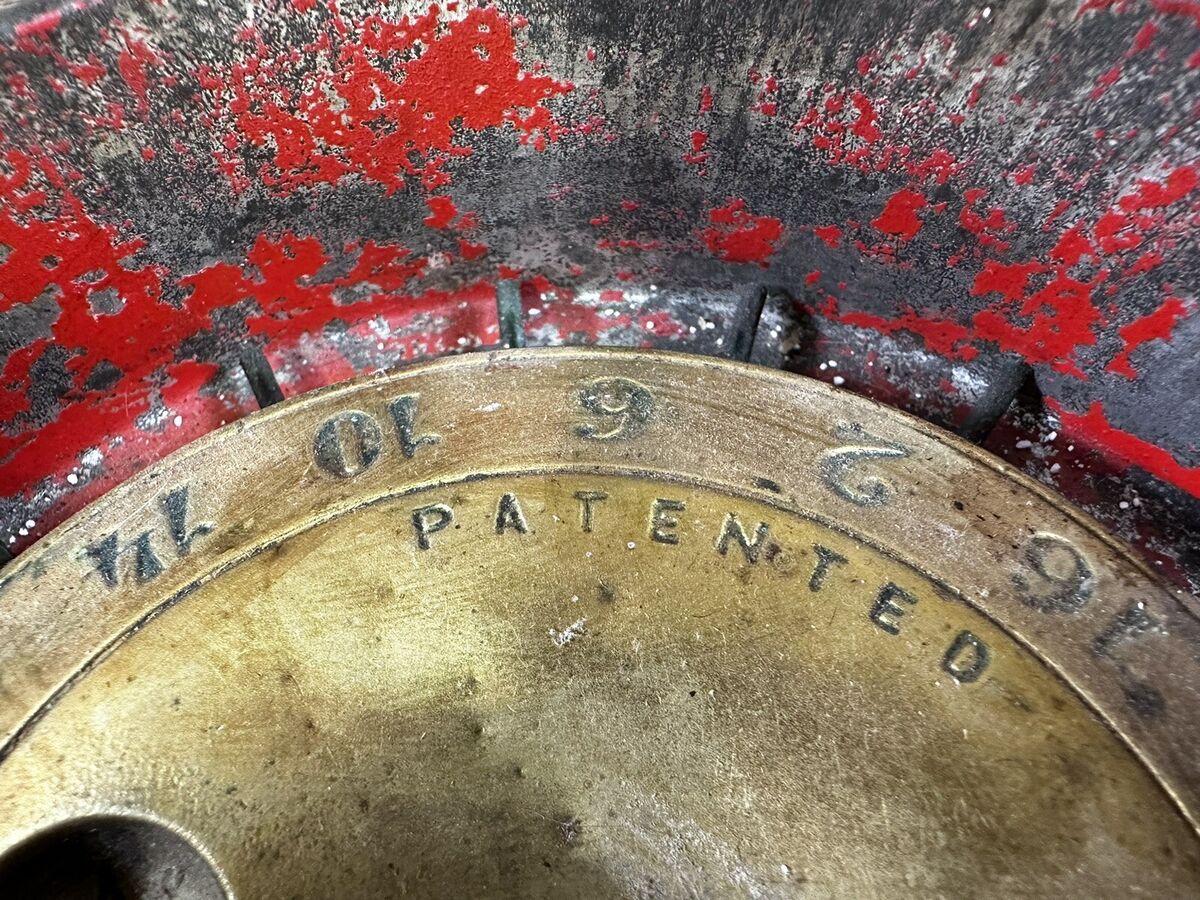This image features a close-up of a metallic mechanism, prominently showcasing a gold, gear-like structure with a half-moon shape. The gold surface is visibly scratched and worn, with black embossed text displaying "969L" and "PATENTED." This section of the mechanism is burnished and old, suggesting significant wear and tear.

Above the gold component, another wheel-like attachment is visible. This upper part appears to have been originally painted red, though much of the paint has chipped away over time, now leaving a mix of black, silver, and some remaining red splotches. This section also includes steel streaks and some reflective areas, indicating a metallic finish underneath the deteriorating paint.

The entire mechanism includes several little black arms or phalanges that extend and curve inward, connecting different parts of the device, creating a complex and worn, yet mechanically intricate appearance.